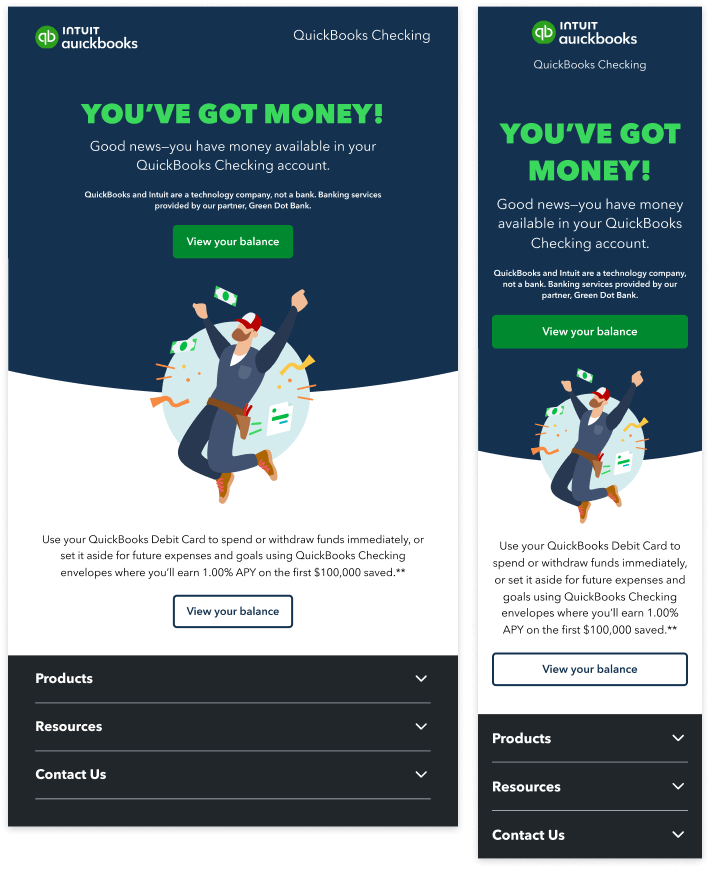This image showcases two Intuit QuickBooks screens, which are nearly identical in layout and content. 

**Left Screen:**
The top half of the left screen features a navy blue background. In the upper right corner, the "Intuit QuickBooks" logo is displayed prominently. Below this, the text "QuickBooks Checking" is visible, followed by a green-font message stating, "You've got money." Beneath this, in white font, the message, "Good news, you have money available in your QuickBooks checking account," is displayed. A green button labeled "View your balance" is positioned under the text. Below this, there is an illustration featuring a man with a red baseball cap and a beard, jumping with his hands in the air. The bottom portion of the screen has a black background with white font options for "Products," "Resources," and "Contact Us," each accompanied by a down arrow indicating the presence of additional information.

**Right Screen:**
The right screen similarly starts with the "Intuit QuickBooks" logo at the top center. Directly below, "QuickBooks Checking" followed by the green-font message, "You've got money," is displayed. The same "Good news, you have money available in your QuickBooks checking account" message appears beneath, accompanied by a green "View your balance" button. The illustration of the man with a red baseball cap and a beard jumping with his hands in the air is also present here. At the bottom, the options for "Products," "Resources," and "Contact Us" are available in white font on a black background, each with a down arrow to access further information.

Both screens emphasize the availability of funds in the QuickBooks checking account and offer consistent navigation options and visual elements.